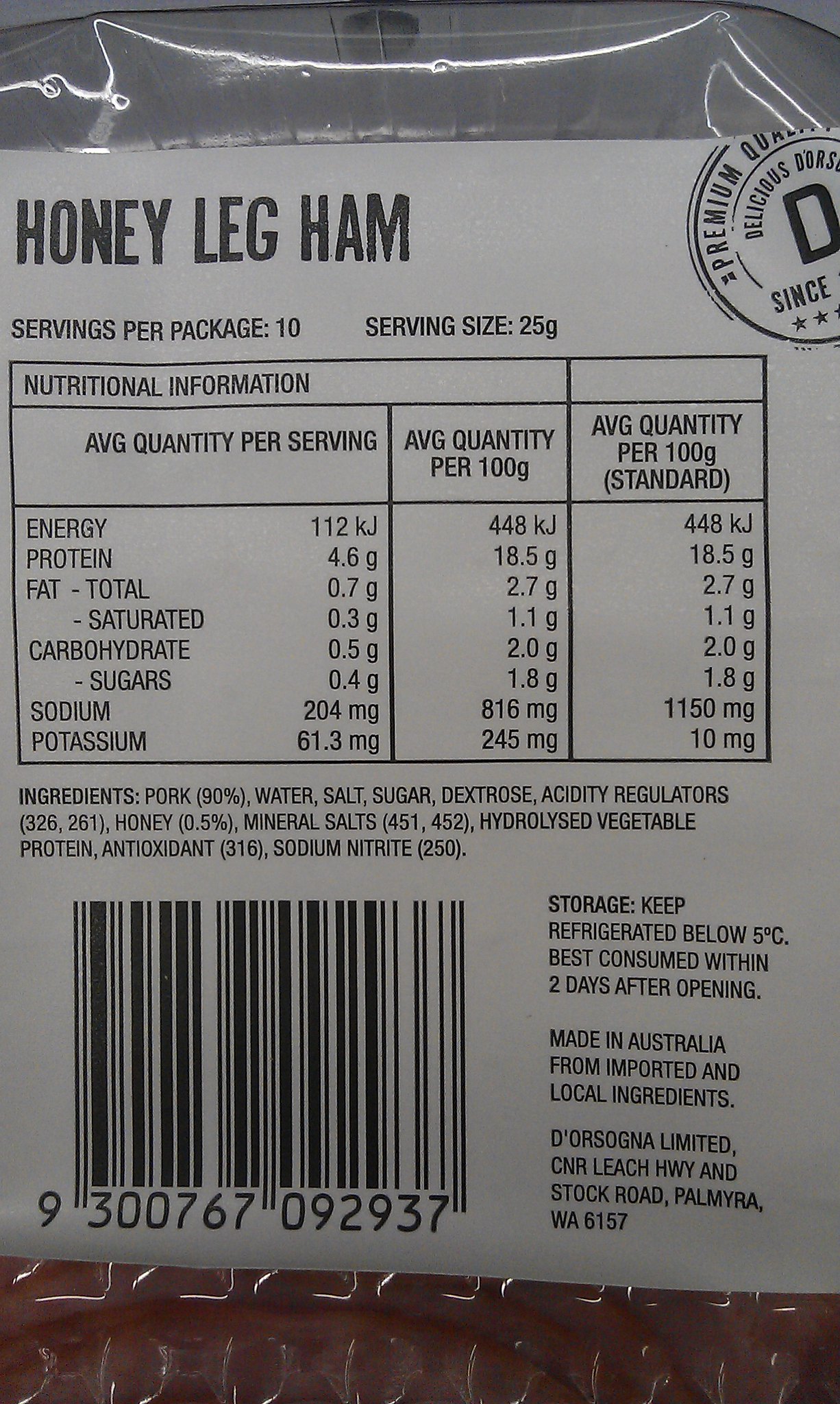This image is a detailed photograph of a label on a honey leg ham package. The packaging consists of clear plastic, with a white label featuring black text. At the top left of the label, in bold letters, it states "Honey Leg Ham." Directly below this, it specifies "servings per package: 10" and "serving size: 25g."

On the right-hand side of the label, there is a partially visible circular design that reads "Premium" and "Delicious" with an incomplete word starting with a "D." The label contains a large rectangular section subdivided into three columns that provide nutritional information. The first column lists the average quantity per serving with values such as Energy 112kJ, Protein 4.6g, Fat 0.7g, Saturated Fat 0.3g, Carbohydrates 0.5g, Sugars 0.4g, Sodium 204mg, and Potassium 61.3mg. The second column details the average quantity per 100 grams, including Energy 448kJ, Protein 18.5g, Fat 2.7g, Saturated Fat 1.1g, Carbohydrates 2.0g, Sugars 1.8g, Sodium 816mg, and Potassium 245mg. The third column repeats the average quantity per 100 grams labeled as standard, showing identical values except Sodium listed as 1150mg and Potassium as 10mg.

Beneath this nutritional information is the ingredients list: Pork (90%), Water, Salt, Sugar, Dextrose, Acidity Regulators (326,261), Honey (0.5%), Mineral Salts (451,452), Hydrolyzed Vegetable Protein, Antioxidant (316), and Sodium Nitrate (250). The bottom left corner of the label contains a barcode, identified as 9300767092937, and on the right side, it provides storage instructions: "Keep refrigerated below 5 degrees C. Best consumed within 2 days after opening," along with the manufacturer’s information: "Made in Australia from imported and local ingredients," and "DIORSOGNA Limited, CNR, Leach, HWY and Stock Road, PALMYRA WA 6157." At the very bottom of the image, part of the ham can be seen through the plastic packaging, showing a reddish shade.